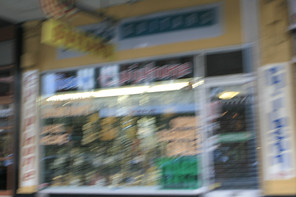This photograph, despite its blurriness and haziness, captures what appears to be a storefront scene or perhaps the interior view of a store looking outward. The composition features multiple advertising signs, including a prominent three-dimensional sign hanging from the ceiling, which likely reads "Guinness," suggesting the sale of beer, possibly in refrigerated sections. A large fluorescent light fixture hangs centrally, illuminating the sales area below. To the right, there's an entrance or exit door, while the walls are painted a creamish yellow hue. Visible merchandise includes sections with green, beige, and blue products, providing a glimpse into the store's diverse offerings.